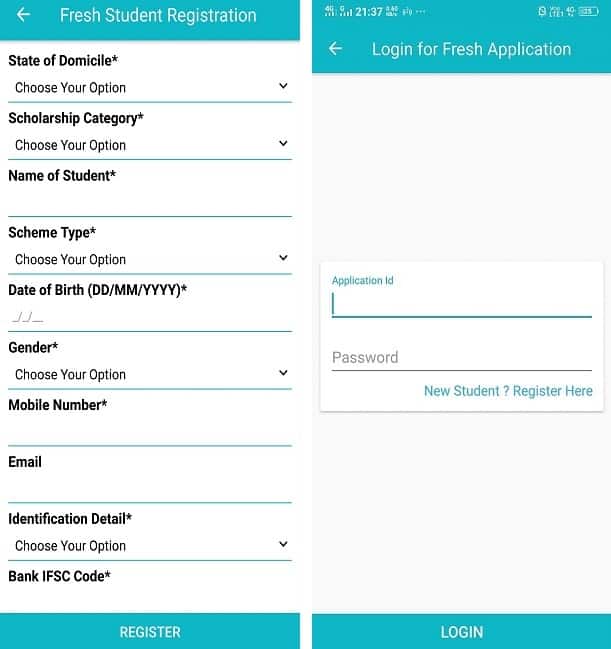This screenshot displays a detailed layout of a student registration page divided into two primary columns, each with distinct features and options.

The leftmost column, highlighted by an aqua green banner at the top, is titled "Fresh Student Registration" in white font. Below this banner, the section lists a series of data entry fields and selection options for students. The first field is labeled "State of Domicile" with a "Choose Your Option" dropdown in black font. The subsequent field, "Scholarship Category," is in bold, followed by another "Choose Your Option" dropdown. Next, a bold "Name of Student" section is left blank for entry, followed by "Scheme Type" with an asterisk and a selection dropdown. The "Date of Birth" field is specified with the format (DD/MM/YYYY) and includes an asterisk, indicating mandatory entry. The "Gender" field, also mandatory, offers a "Choose Your Option" dropdown. Fields for "Mobile Number" and "Email" follow, both of which are blank and filled out by the user. The "Identification Detail" field also provides a dropdown option, and the last field in this column is for entering the "Bank IFSC Code," marked with an asterisk. A blue horizontal line underlines each section indicating where the input or selection appears. At the bottom, a blue banner in all caps white font states "REGISTER."

The second column features a blue banner at the top, displaying the current time (21:37) on the upper left, along with icons presumably indicating network availability and signal strength. On the upper right, there is a bell icon with a slash through it, suggesting notifications are turned off, and a battery symbol showing approximately 60% charge. Below the banner, the section titled "Login for Fresh Application" is displayed in white lettering with a white arrow pointing to the left. This section has a lighter gray background with a white box in the center. The box includes "Application ID" in green font with a green line below it, followed by "Password" in light gray font with a matching light gray line. At the bottom of the white box, the text "New Student? Register here" appears in green font, indicating a link or prompt for new users to register.

This comprehensive caption provides a detailed view of the student registration interface, capturing all elements and formatting for better understanding and navigation.